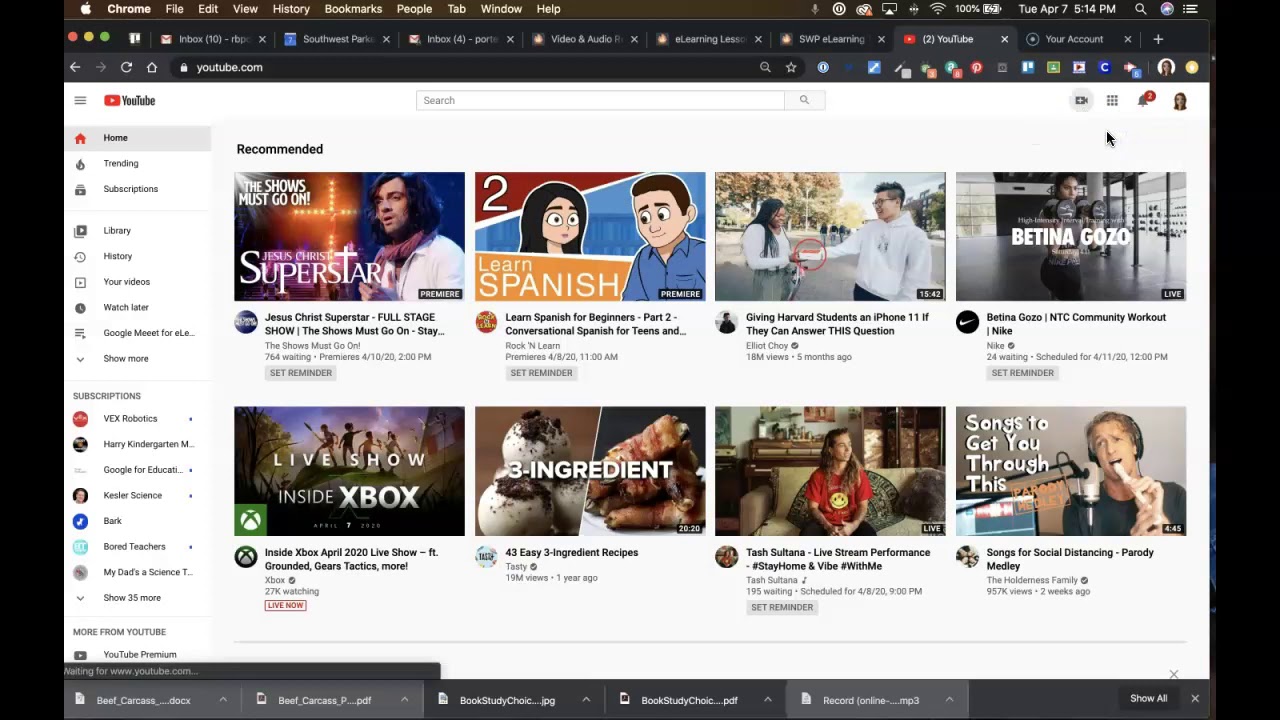This screenshot of the YouTube website captures a typical user interface experience. At the top, the standard browser bar is visible, displaying the YouTube logo prominently. On the left side, a vertical menu includes options such as Home, Trending, Subscriptions, Library, History, and other categories. Directly underneath these, the user’s personal subscriptions are listed.

The central section of the screenshot showcases a variety of recommended videos. The first recommendation is a thumbnail for "Jesus Christ Superstar, Full Stage Show." Following this, a thumbnail for a video titled "Learn Spanish" is displayed. Next, there is a small image that reads, "Giving Harvard Students an iPhone 11...If They Can Answer This Question." To the right of that, another selection features "Bettina Gozo, NTC Community Workout."

Below these recommendations, another row of suggested content is visible. It begins with a live show titled "Inside Xbox" and is followed by a video labeled "43 Easy, Three-Ingredient Recipes." Next in the lineup is a live stream performance, and finally, a video titled "Songs to Get You Through This" appears.

This comprehensive screenshot exemplifies YouTube's interface and the diverse content it offers to users.